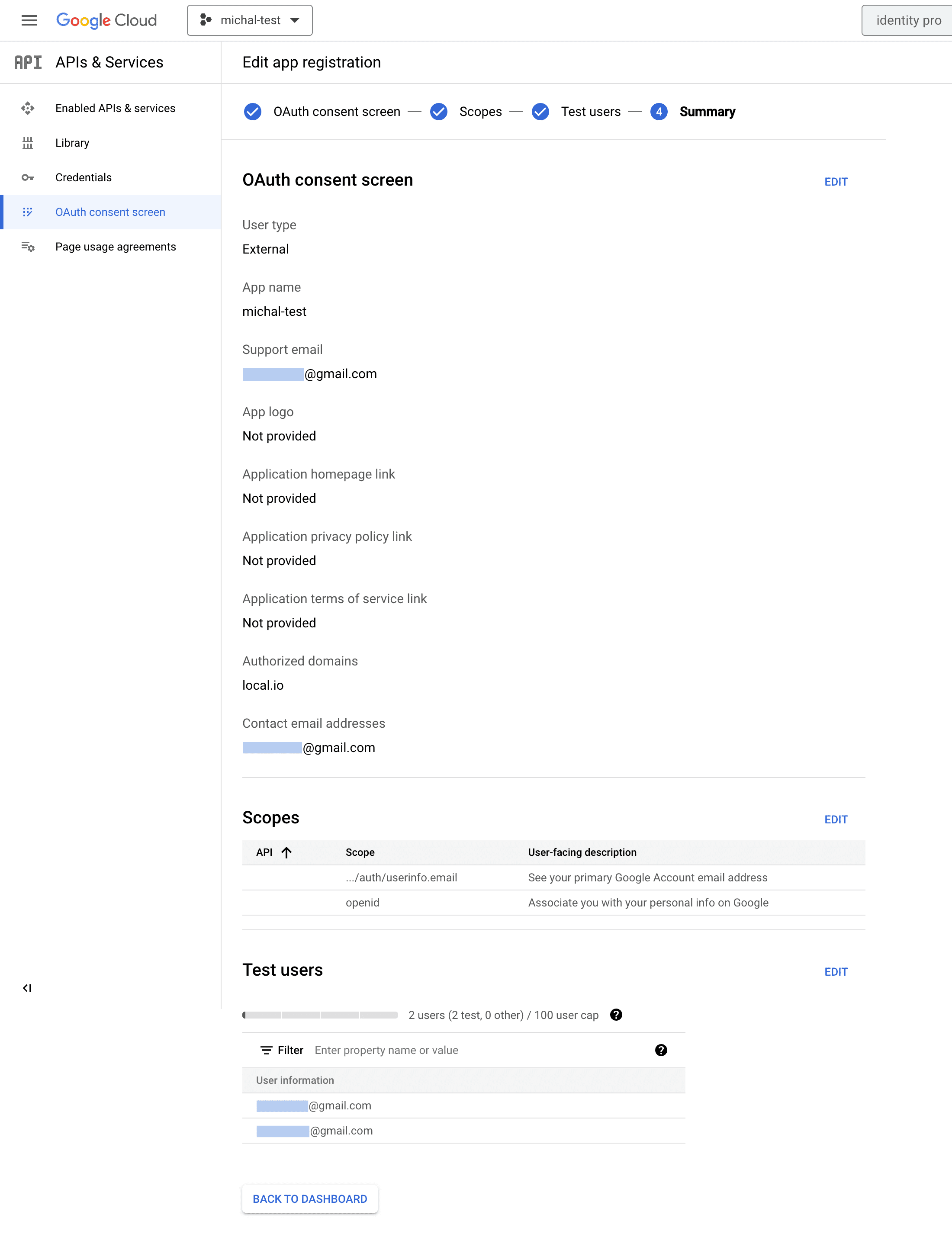The image displays a detailed view of the Google Cloud interface. Centered at the top-left corner, "Google Cloud" is prominently labeled. Below this header, the left-hand navigation pane lists various subcategories under "APIs & Services," including "Library," "Credentials," "OAuth consent screen," and "Page usage agreements."

The main section of the interface is dedicated to editing an app’s registration details, starting with a header that reads "Edit App Registration." Directly beneath this, tabs for "OAuth Consent Screen," "Summary," and "Test Users" are displayed, each marked by a circle with a check mark indicating their status.

The "OAuth Consent Screen" tab is active, presenting various fields related to user consent and app registration. Details include:

- **User Type:** External
- **App Name:** Michael Test

Following this, several fields indicate whether particular pieces of information are provided:
- **Support Email:** [Crossed out]@gmail.com (indicating the beginning part of the email is redacted)
- **App Logo:** Not Provided
- **Application Home Link:** Not Provided
- **Application Privacy Policy Link:** Not Provided
- **Application Terms of Service Link:** Not Provided

Further down, the section labeled "Authorized Domains" lists "Local.io," while another segment for "Contact Email Addresses" shows a partially redacted email, [Blanked Out]@gmail.com. 

The "Scopes" section outlines specific permissions and access levels, though text details are hard to discern. Finally, the "Test Users" section lists two email addresses, both with the first part obscured by blue bars indicating redaction:
- [Blank]@gmail.com
- [Blank]@gmail.com

Each "Blank" placeholder represents redacted portions of email addresses, ensuring privacy. The interface overall provides a comprehensive snapshot of the user’s configuration and registration details within the Google Cloud platform.